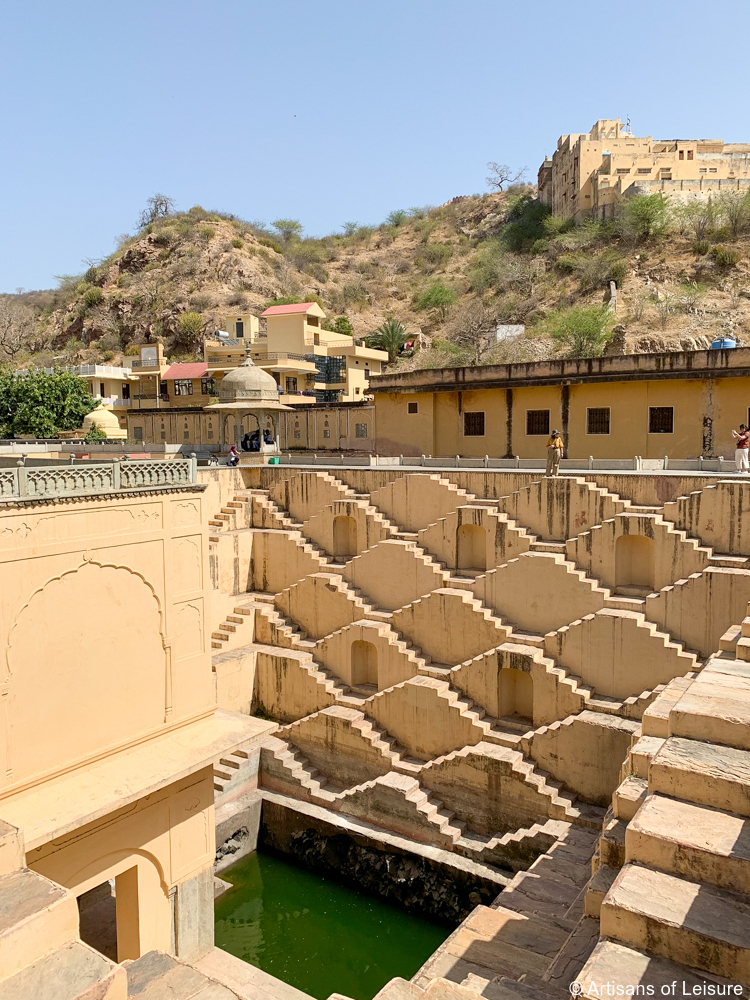Here is a refined and detailed caption for the image:

"In this captivating image, a sprawling, multi-floored adobe fortress commands attention in the foreground, distinguished by its light brown hue and intricate architectural design. The fortress, standing at least five stories tall, encloses a dark green, stagnant pool at its center, resembling a large, unchlorinated swimming pool. A sturdy wooden roof crowns the upper floors, shading the tiers of stairways that descend gracefully to the pool level. The fortress is encapsulated by a protective wall on its lower right quadrant, enhancing its imposing appearance.

In the upper right corner, a smaller but equally striking brown adobe fortress perches atop a hill, its presence accentuated by the pristine blue sky that serves as a serene backdrop. This hill extends diagonally towards the left, creating a sense of depth and continuity in the landscape, matched by a smaller hill on the left side of the image.

The composition is a stunning interplay of natural and man-made elements, with the fortresses harmoniously set against the lush hillside and the clear expanse of sky, evoking a sense of timeless beauty and historical grandeur."